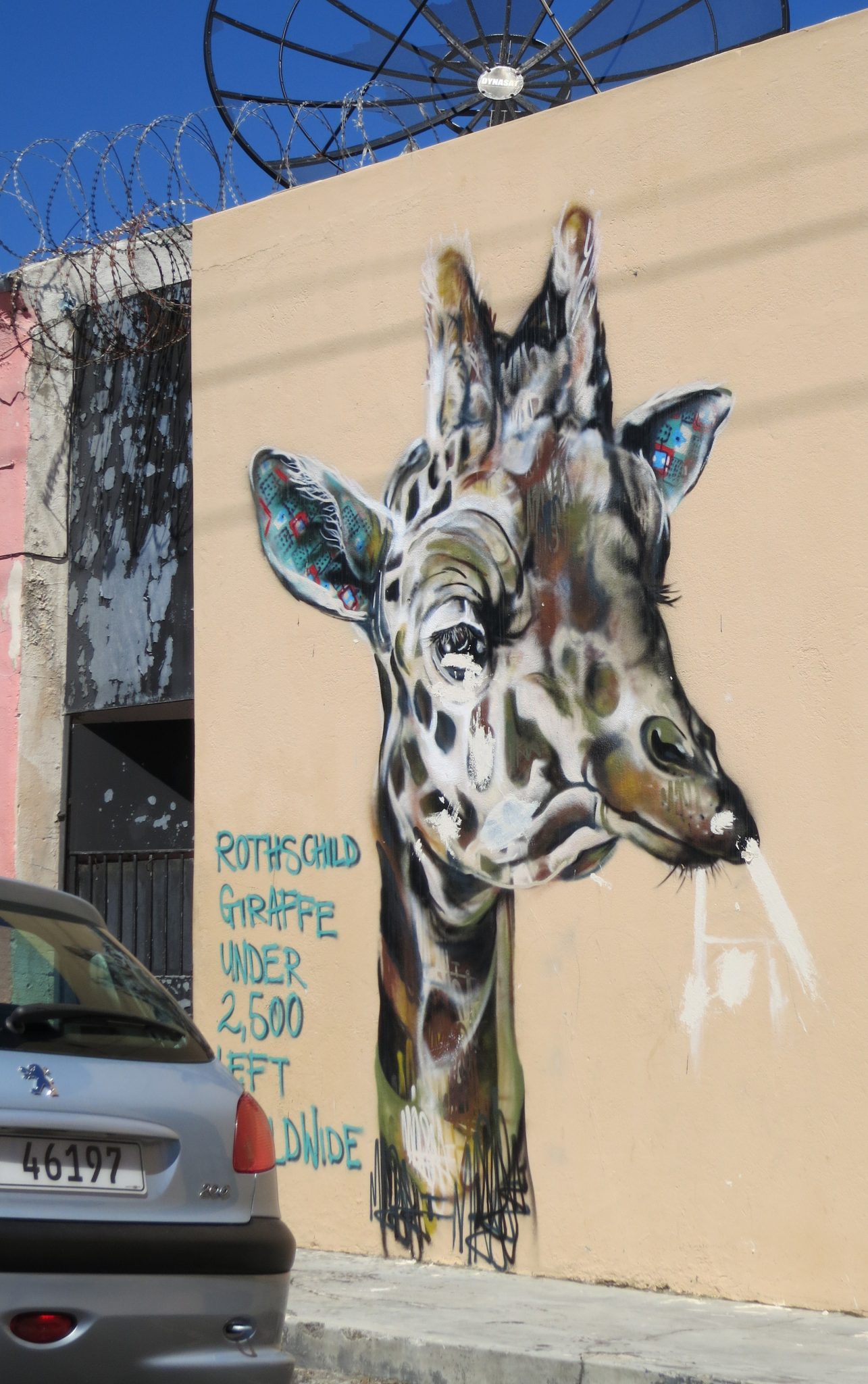This image captures a vivid street scene dominated by a graffiti mural of a Rothschild's giraffe. Painted on a large beige wall, the giraffe's expressive, slightly sad face takes up most of the mural, exhibiting a mix of brown, beige, blue, and greenish textures. The giraffe appears to be blowing air out of its nose, creating a dynamic sense of movement with the white strokes around its nostrils. Accompanying the mural is text in an aqua or teal color reading, "Rothschild Giraffe under 2500 left worldwide," highlighting the endangered status of this species. 

In the foreground, a gray European car with a license plate number 46197 is parked at the curb. The sidewalk in front of the mural leads to a building entryway to the left, which is black and flanked by a pink wall. Coiled razor wire adorns the roof edges and the area above the entrance, adding a gritty, urban feel to the scene. A satellite dish is perched atop the building, contributing to the complex background. Despite some chipping in the mural, particularly around the eyes, cheeks, and nose, the image poignantly underlines the mural's activist message while encapsulating the character of the urban environment.